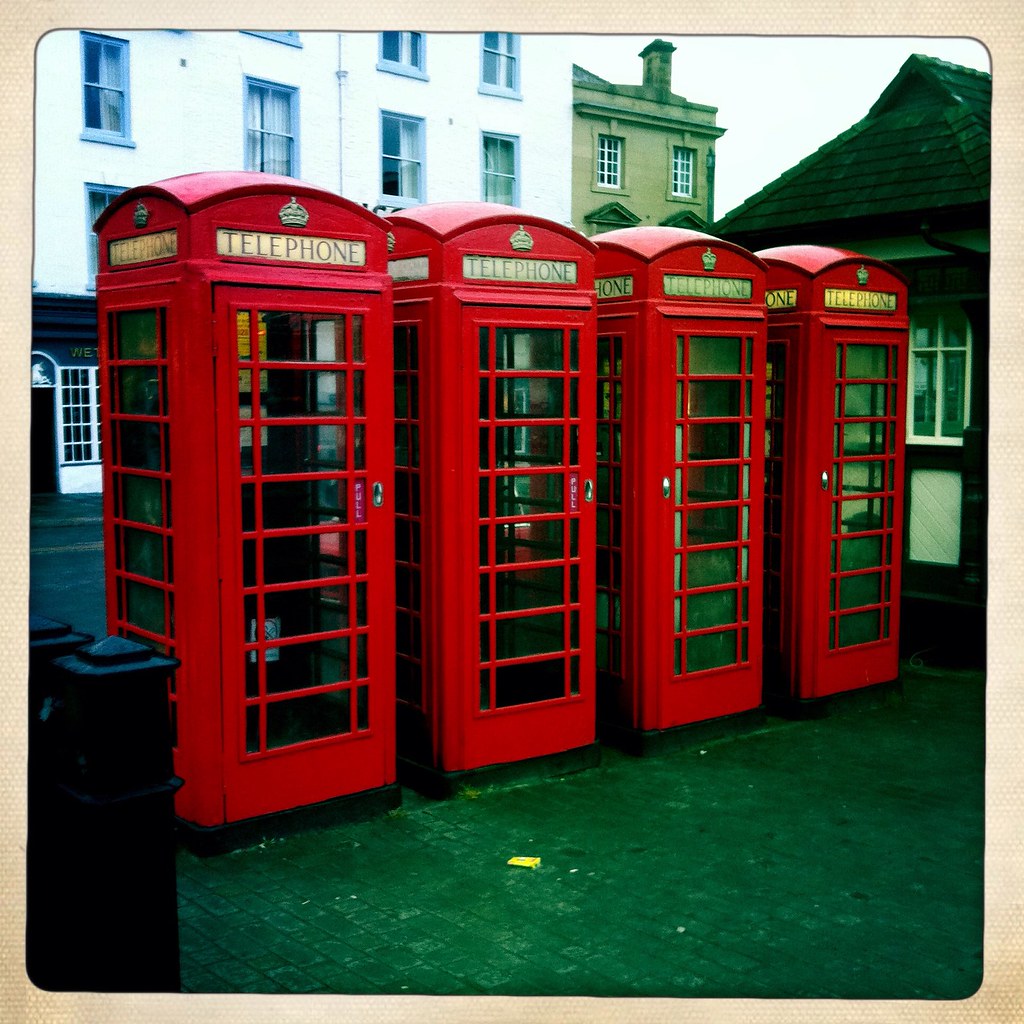This photograph features four iconic British red telephone booths standing tall in a row, reminiscent of those found in London, England. Each booth displays the word "TELEPHONE" at the top, crowned with a small golden emblem, and features glass windows with wooden dividers painted to match the vibrant red exterior. The roofs are elegantly arched, with one of the booths illuminated from within. The booths are situated on a brick-paved sidewalk, flanked by metal posts likely intended to prevent vehicular collisions. In the background, a residential street is visible, lined with historic buildings including a multi-story white structure, a gray house with a chimney, and a lower brown building accented with white windows. A yellow object lies discarded on the ground in front of the booths, adding a minor touch of urban imperfection to the scene.